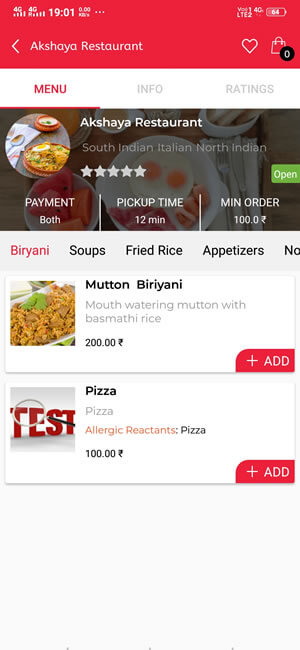An image of a smartphone screen showcasing a restaurant app interface. At the top of the screen, the status bar displays several icons: signal strength showing 4 bars with '424G', the time '19:01', an icon indicating 0.0 KB data usage, and three dots suggesting additional settings. Further to the right are icons showing 'VOLTE', '4G', and the battery level at 64%.

Below the status bar, on a red background, there are navigation elements: a left arrow labeled 'Akshaya Restaurant' on the left side and icons of a heart and a shopping bag on the right side. A navigation bar on a white background shows four tabs: 'Menu', 'Info', 'Ratings', with 'Menu' being highlighted and underlined in red.

The main section features an image of various food items on plates, including eggs, watermelon, vegetables, and another dish with rice and eggs. At the top center of the image, the text reads "Akshaya Restaurant," followed by "South Indian, Italian, North Indian," and a 5-star rating.

Below the main image, in a section for order information, the text reads "Payment: Both | Pickup time: 12 minutes | Min order: 100 [unrecognized currency symbol]."

Further down, a menu list includes items such as 'Biryani' (highlighted in red), 'Soups,' 'Fried Rice,' and 'Appetizer' (all in black). The first menu item, 'Mutton Biryani,' is described as "Mouthwatering Mutton with Basmati Rice," priced at '200.00 [currency symbol].' To the left of this description is a picture of a white bowl filled with brown rice and garnished with two leaves. The bottom right corner of this item features a red 'plus' add button.

Another menu item, 'Pizza,' is described as "Allergic Reacting Pizza," priced at '100.00 [currency symbol].' To the left, there is an image of a white background with red text saying "Test," magnified by a magnifying glass. This item also has a red 'plus' add button at the bottom right corner.